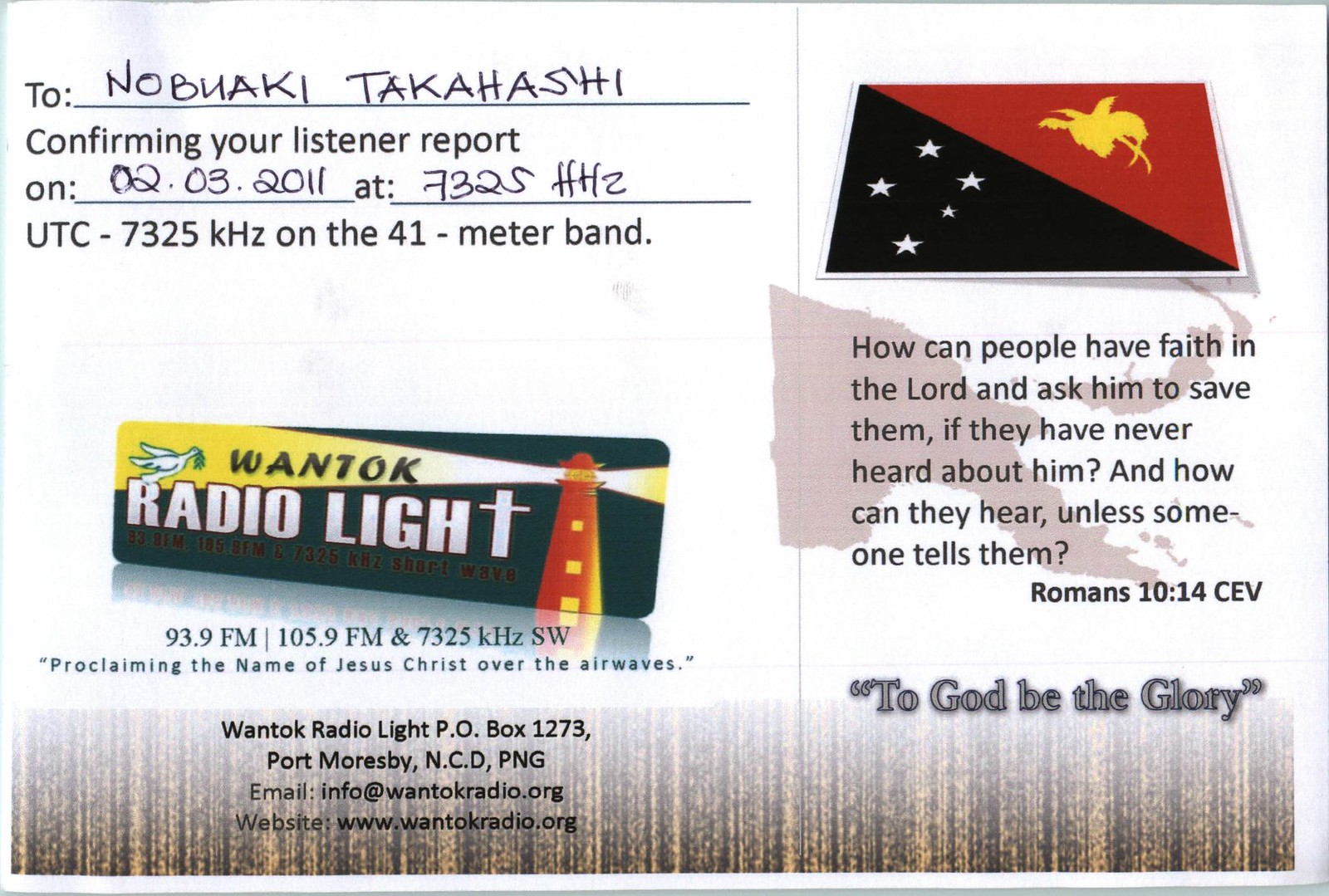The image depicts a confirmation card with a white background from Wontok Radio Light, indicating receipt of a listener report. Addressed to Nobuaki Takashi, it confirms a report on 02-03-2011 at 7325 HHZ, UTC 7325 KHZ on the 41-meter band. The card features the station information, including frequencies 93.9 FM, 105.9 FM, and 7325 KHZ SW, emphasizing its mission of "proclaiming the name of Jesus Christ over the airwaves." The Wontok Radio Light logo, a lighthouse with light beams, is prominently displayed. The address is listed as PO Box 1273, Port Moresby, NCD, PNG. Contact details include an email (info@wontotalkradio.org) and a website (www.wontotalkradio.org). To the right, there's a flag of Papua New Guinea, bisected diagonally with the bottom left in black housing five white stars, and the top right in red with a yellow bird of paradise. Below the flag, a Romans 10:14 quote reads, "How can people have faith in the Lord and ask him to save them if they have never heard about him? And how can they hear unless someone tells them?" followed by, "To God be the glory."